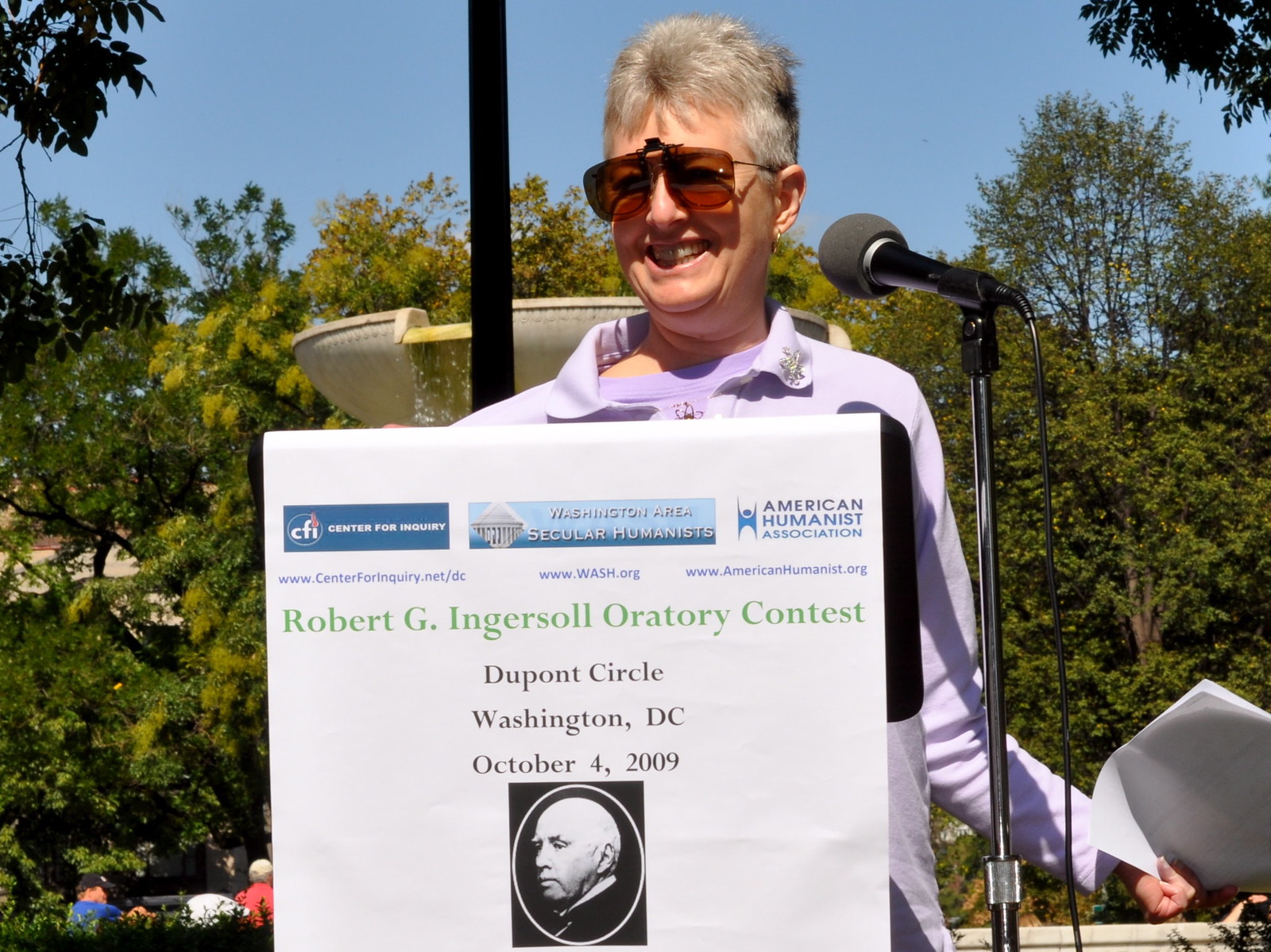In a sunlit park under a clear blue sky, an older woman with short gray hair and large brown-tinted sunglasses stands at a thin podium. Flashing a big smile that shows her teeth, she is elegantly dressed in a purple top layered with a white or light purple shirt and gold earrings. A black microphone on a stand is positioned off to her right, while she holds several sheets of paper in her left hand. Her right hand is concealed by a large white sign affixed to the podium. The sign prominently advertises the "Robert G. Ingersoll Oratory Contest" in green letters, along with "DuPont Circle, Washington, D.C., October 4, 2009" in black letters. There is an old-timey black and white portrait of a man, likely Robert G. Ingersoll, centered on the poster. Behind her are tall green trees, a few people sitting on benches, and the serene ambiance of an outdoor gathering.